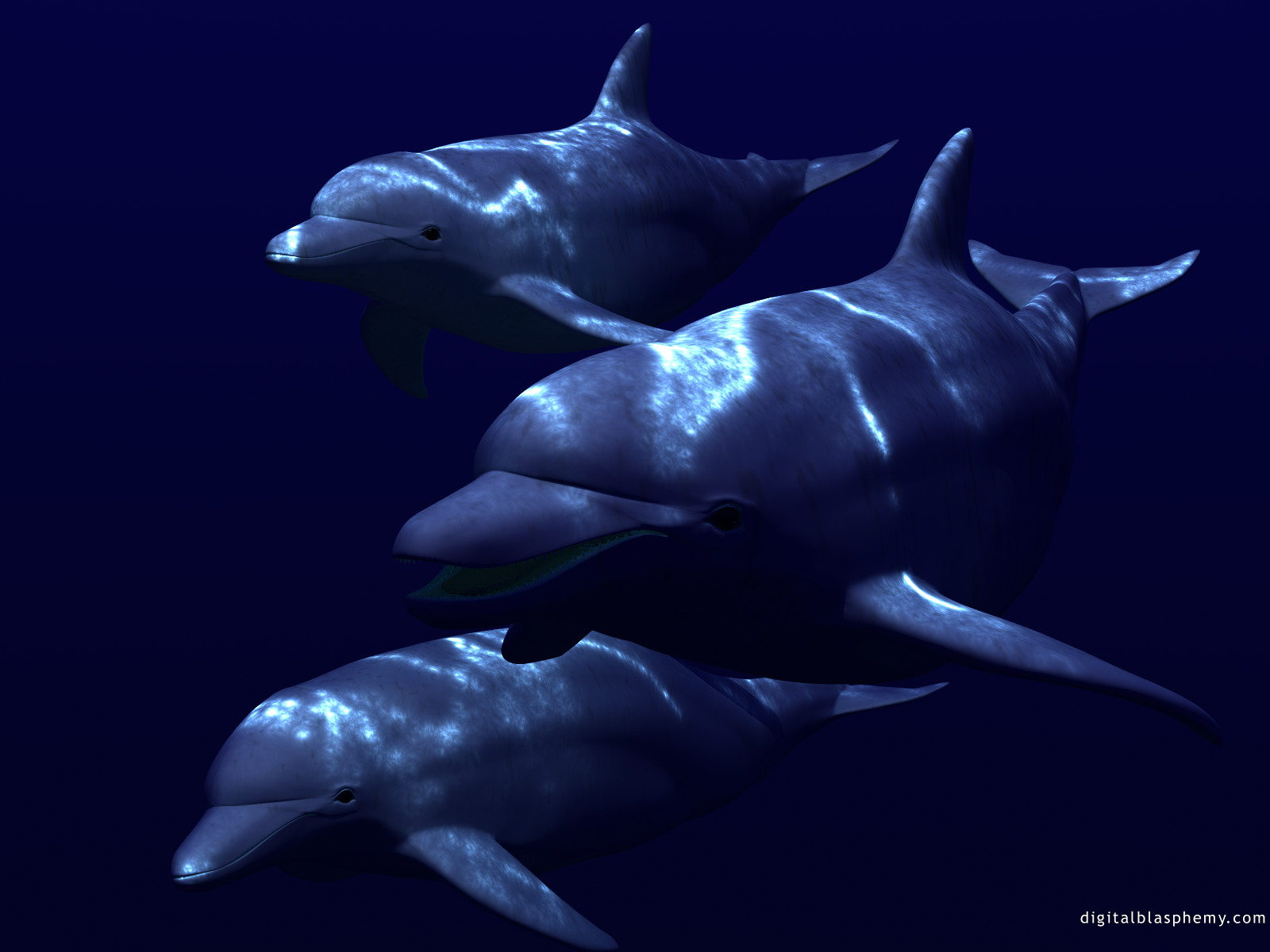The image depicts an underwater scene featuring three dolphins swimming in dark, blue water. Each dolphin, with their characteristic two pectoral fins on the sides and a back fin, along with a tail fin, is bathed in light shining from the surface above. The dolphin closest to the camera, positioned centrally, has its mouth open, while the other two, one positioned above and the other below, have their mouths closed. The dolphins' bodies exhibit a bluish-gray hue, enhanced by shimmering light that creates white splotches and streaks on their backs, simulating the effect of sunlight filtering through the water. The overall effect is a striking pattern of light and dark, with the dolphins almost appearing to glow against the dark backdrop. The bottom right-hand corner of the image contains the text "digitalblasphemy.com," indicating the creator of the image.